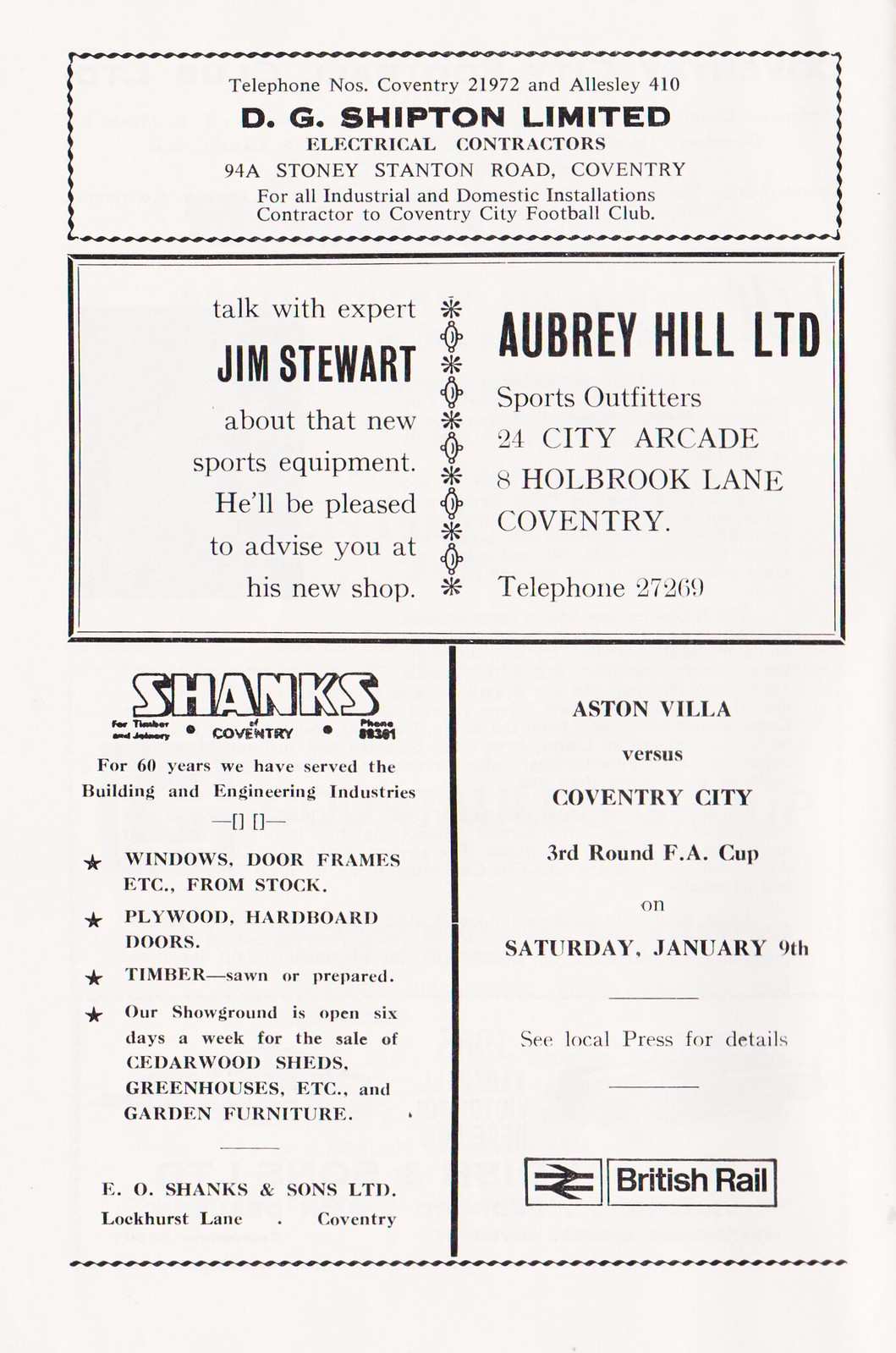This image features the front cover of a soccer program on a white card. At the top, there are two horizontally aligned rectangles. The first smaller rectangle, outlined with black dotted lines, contains the text, "Telephone Number Coventry 21972 and Allisay 410-DG Shipton Limited Electrical Contractors, 948 Stony Stanton Road, Coventry, for all industrial and domestic installations. Contractor to Coventry City Football Club." Beneath it, a larger rectangle holds two sections. The left column reads, "Talk with expert Jim Stewart about that new sports equipment, he'll be pleased to advise you at his new shop. Aubrey Hill Sports Outfitters, 24 City Arcade, 8 Hallbrook Lane, Coventry, Telephone 27269." The right side mentions symbols and additional text in bold.

Below these, on the left side, there is a vertical rectangle for D.G. Shanks and Sons Limited, reading, "Shanks Coventry. For 60 years we have served the building and engineering industries: windows, doors, frames, etc. from stock. Plywood, hardboard, doors, timber, sawn or prepared. Our show ground is open six days a week for the sale of cedar, wood sheds, greenhouses, etc. and garden furniture. F.O. Shanks and Sons Limited, Lockris Lane, Coventry." Adjacent to this, on the right, another vertical rectangle announces, "Aston Villa vs. Coventry City. Third round FA Cup on Saturday, January 9th. See local press for details." with British Rail branding at the bottom.